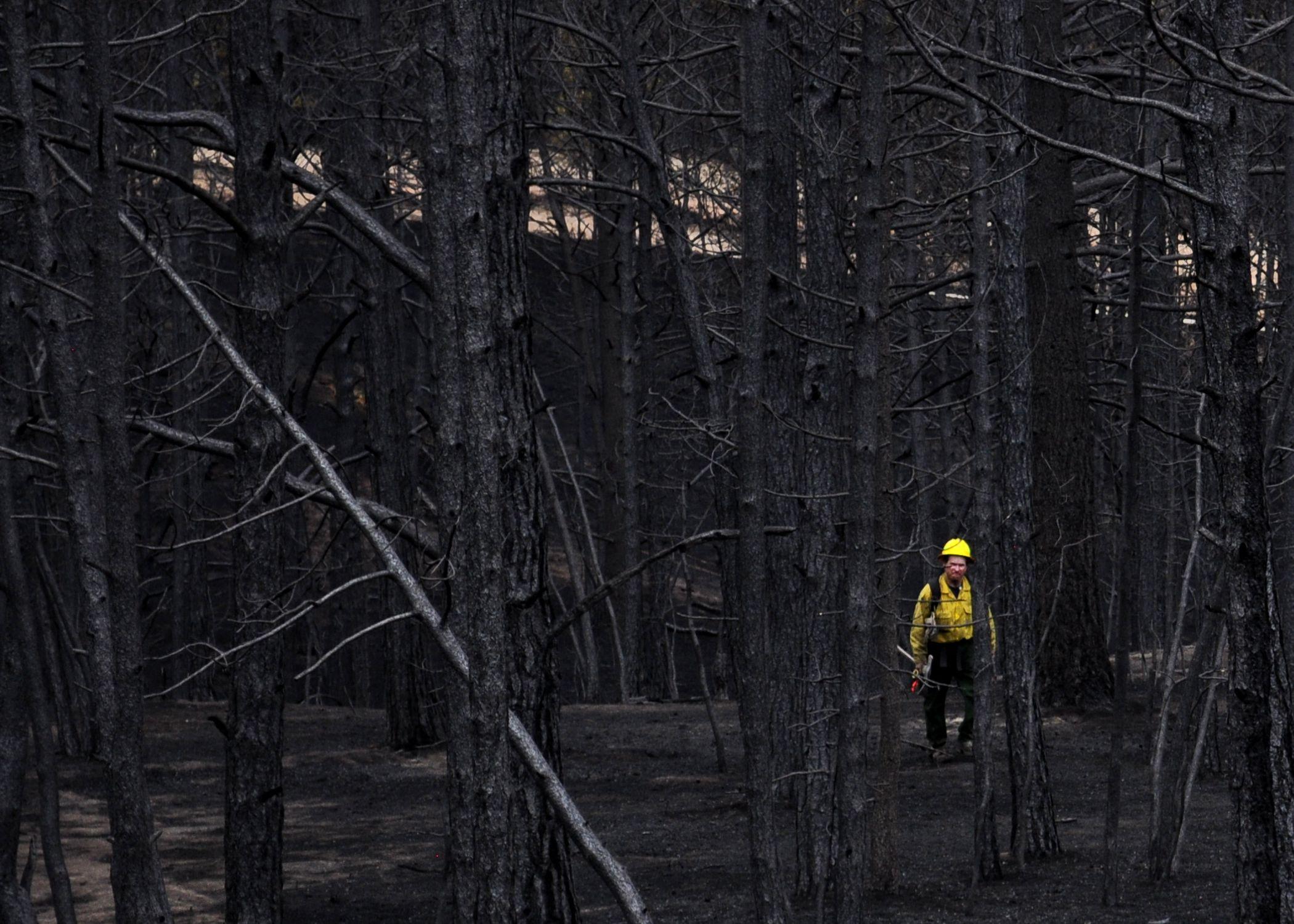The photograph depicts a cloudy, potentially winter day in a dense forest with numerous tall, branchless tree trunks predominant in the scene. The ambiance is dark and slightly gloomy, accentuated by the white sky visible through the trees and the scattered white patches on the ground, suggesting either snow or a clearing. Prominently on the lower right-hand side, a man stands out, dressed in black pants, a yellow jacket, and a yellow hard hat, along with a black strap extending across his torso, possibly from a backpack. He appears to be holding an indistinct object which could resemble either a tool or a piece of equipment. Surrounding him, the forest floor is littered with fallen branches and needles, adding to the desolate wintery landscape. The man's attire and the object in his hand suggest he may be a worker, possibly in the process of restoring power or conducting forest maintenance.